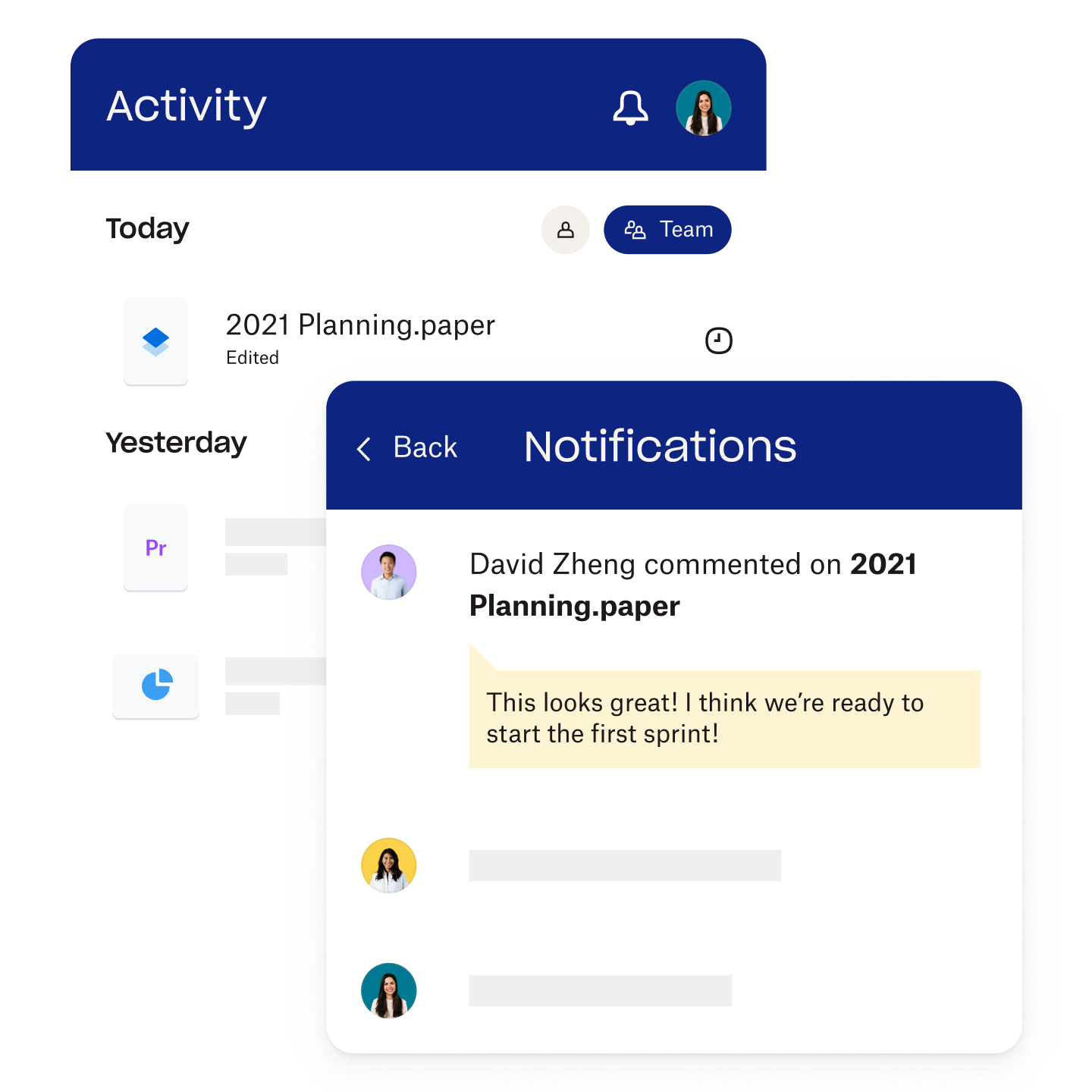In the image, we see a digital workspace where the team is actively engaged in planning for 2021. The screen showcases a document titled "2021 Planning Paper," which appears to be the main focus of the meeting. A notification overlay is visible on the left side, noting that David Zhang has commented on the planning paper, stating, "This looks great. I think we're ready to start the first sprint."

The layout of the interface reveals some design details: the notification area, which has a blue highlight, contrasts with the predominantly white background of the rest of the screen. In the top right corner, there's a small circular profile picture of a team member, who is wearing a shirt, likely indicating the active user. Similarly, in the bottom section of the screen, another small circular profile picture of another team member in a shirt is displayed. Both these profile pictures add a personal touch to the digital workspace, assuring the presence and participation of team members in this crucial planning phase.